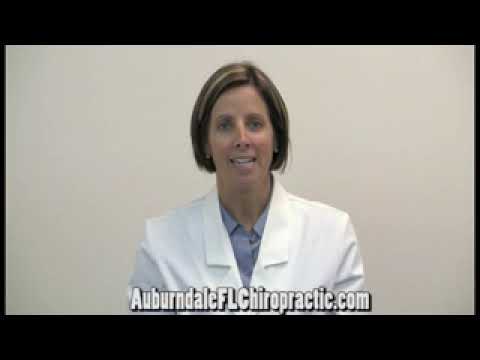The image depicts a woman, likely in her late 30s, who appears to be a chiropractor, based on her attire and the context provided. She has short, brown hair with some blonde streaks and a neutral, serious expression on her face. She is dressed in a white lab coat with a blue-collared shirt underneath. The background is a plain, light color—either white or beige. At the bottom of the image, there is a website URL, "auburndaleflchiropractic.com", written in white text bordered by black horizontal strips. This suggests that the image might be a screenshot from a video, potentially a commercial or instructional content for a YouTube channel related to chiropractic services.